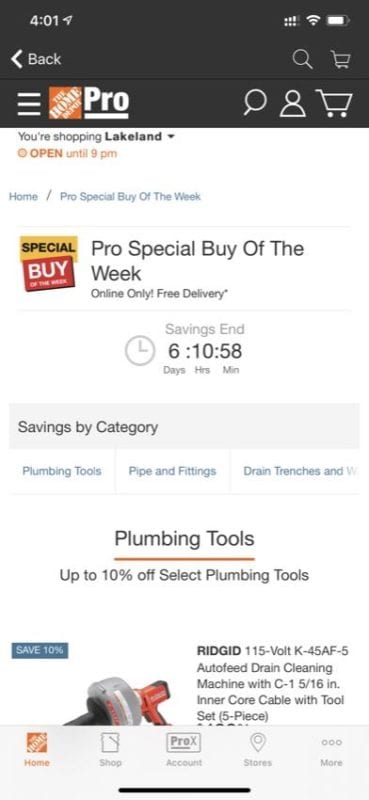**Detailed Caption:**

On a mobile phone display, the Lakeland shopping website headline announces that the store is open until 9 PM. A prominent feature of the page is the "Special Buy of the Week," available exclusively online with free delivery. This week's highlighted deal is on plumbing tools with discounts of up to 10% on selected items. Featured prominently is an image of an auto-feed drain cleaning machine equipped with a C-1 5/16-inch inner core cable and a five-piece tool set. Within this promotional category, there are clickable headings for "Plumbing Tools," "Pipe and Fittings," and "Drain Trenches." A countdown timer indicates that the savings will end in 6 days, 10 hours, and 58 minutes, urging customers to act quickly to take advantage of these special offers.